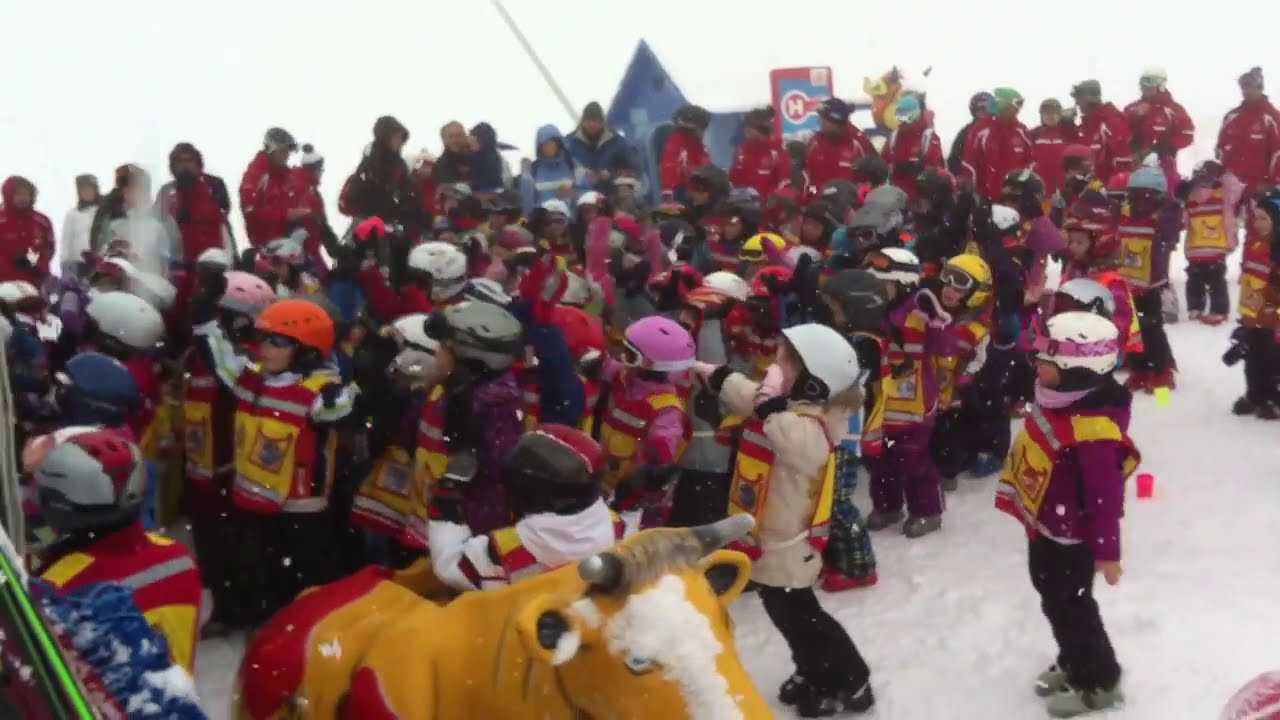In this outdoor, daytime winter scene, a group of children, around 5 or 6 years old, are gathered on a snowy terrain, dressed warmly in jackets, pants, and a mix of helmets—white, pink, and red. The children stand in profile, looking towards the left, with the cloudy sky and a snowy ground setting the backdrop. In the foreground, there is a vibrant red and blue sculpture or stuffed figure resembling a cow. Surrounding the children, a group of adults, potentially parents, in red ski jackets, stands in a row. In the background, amid the snowy setting, a sign with the letter "H" is visible, adding a touch of detail to this wintery scene. The scene is accentuated with colors such as white, red, blue, gray, yellow, pink, and orange, creating a vivid and cheerful atmosphere.